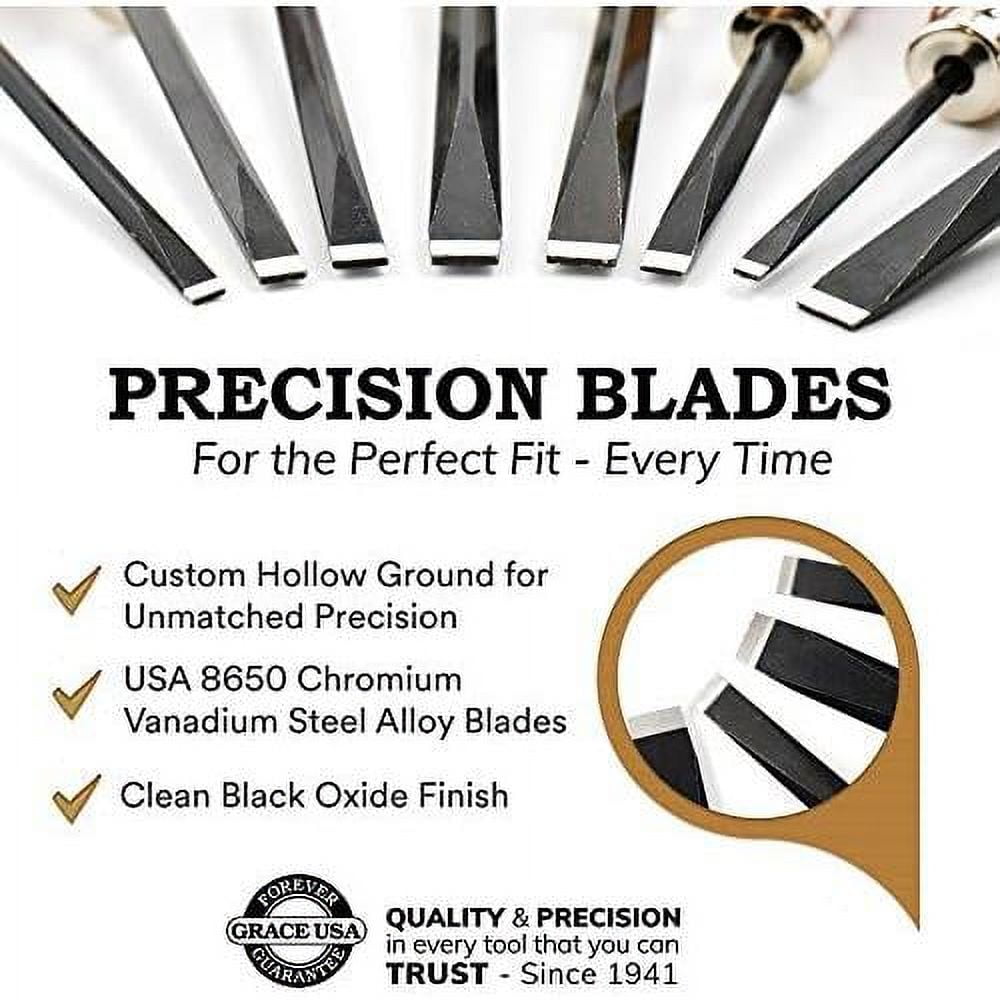This advertisement features an array of precision blades, prominently highlighting their superior quality and design. At the top of the image, there is an arching display of eight sleek, black blades with varying widths from left to right, each tipped with a distinctive white horizontal line. Below this display, bold black text reads “Precision Blades” followed by the tagline, "For the perfect fit - every time."

Further down, three bullet points detail the key attributes of the blades: "Custom hollow ground for unmatched precision," "USA 8650 chromium vanadium steel alloy blades," and "Clean black oxide finish." To the left of this text, there is a yellow box with an inset image of the blades under a magnifying glass. To the right, a small yellow circle featuring a round panel is visible. Additionally, the ad includes a trademark emblem—a black circle with white writing. Surrounding an oval that says "Grace USA," it reads “Forever Guarantee” and “Quality and precision in every tool you can trust since 1941.”